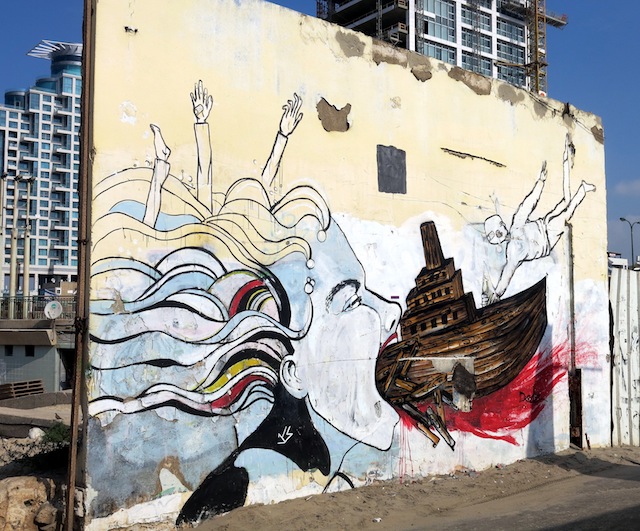The image depicts a detailed and somewhat surreal mural painted on the peach-colored wall of a building that looks like it's in a run-down part of town, possibly where another building was demolished. The focal point of the mural is the profile of a woman's face, rendered in stark white with her mouth dramatically wide open. Her flowing hair, bursting with multicolored streaks including black, green, yellow, red, pink, blue, and white, streams behind her. Emerging from her hair are various human body parts, such as a foot and two arms, suggesting people are entwined within it. The woman's mouth is consuming a large wooden ship, which is halfway inside. The front of the ship appears damaged, with splintered wood and red, blood-like marks emanating from her mouth, adding a gory touch. Additionally, more body parts appear under the ship, further enhancing the eerie, chaotic scene.